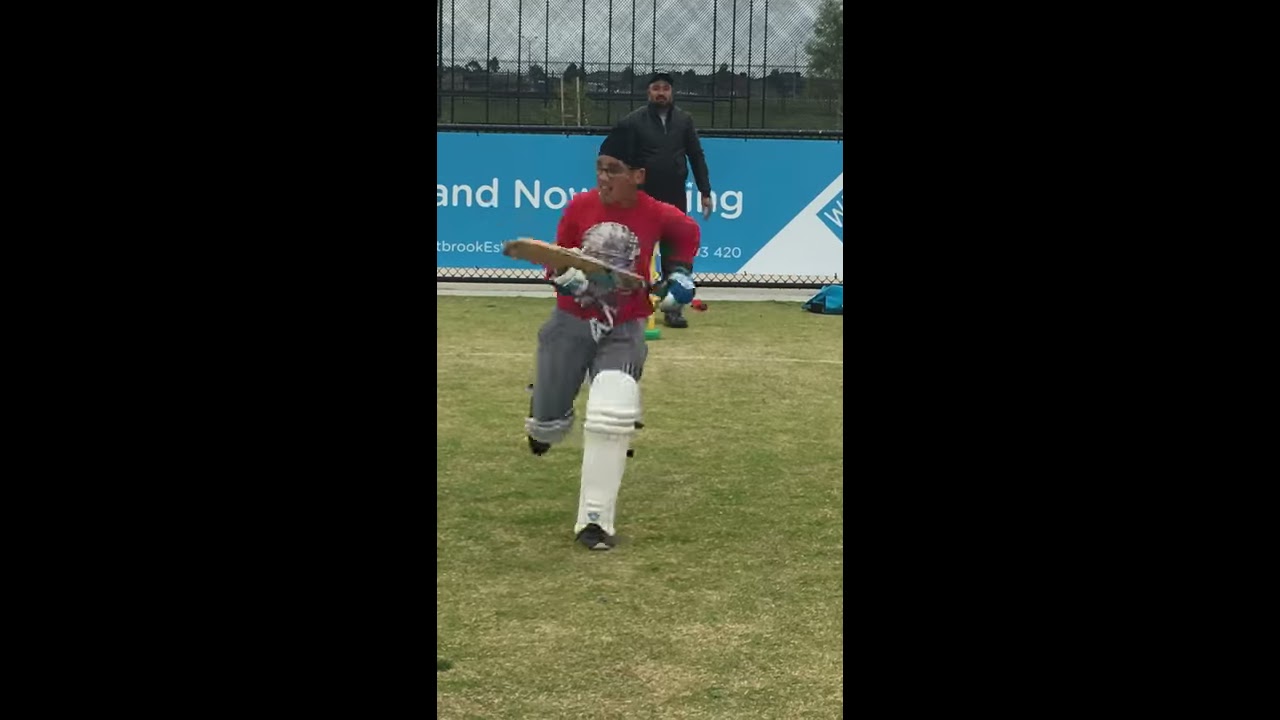The image captures a lively scene set on a green grass field, possibly during a sports game, framed by a black border. At the center, a young boy, likely of Indian descent, is captured mid-run. He wears a long-sleeved red shirt adorned with a white logo, gray sweatpants, and white shin guards extending from his knee to his ankle. His attire includes blue and white padded gloves, a black headband, and black plastic glasses. In his hands, he holds a cricket bat, suggesting he is actively playing the sport. The boy's darker-colored skin tone and expressive motion add life to the scene. Positioned slightly behind the boy, towards the top of the image, stands an older man, potentially a coach. The man is dressed in a blue zip-up jacket, black baseball cap, and black shoes, observing the boy's actions. The background features a light blue and white billboard, which remains partially illegible, hinting at a sports advertisement or announcement. This vivid image, set outdoors in daylight, captures the energetic essence of a cricket game in progress.